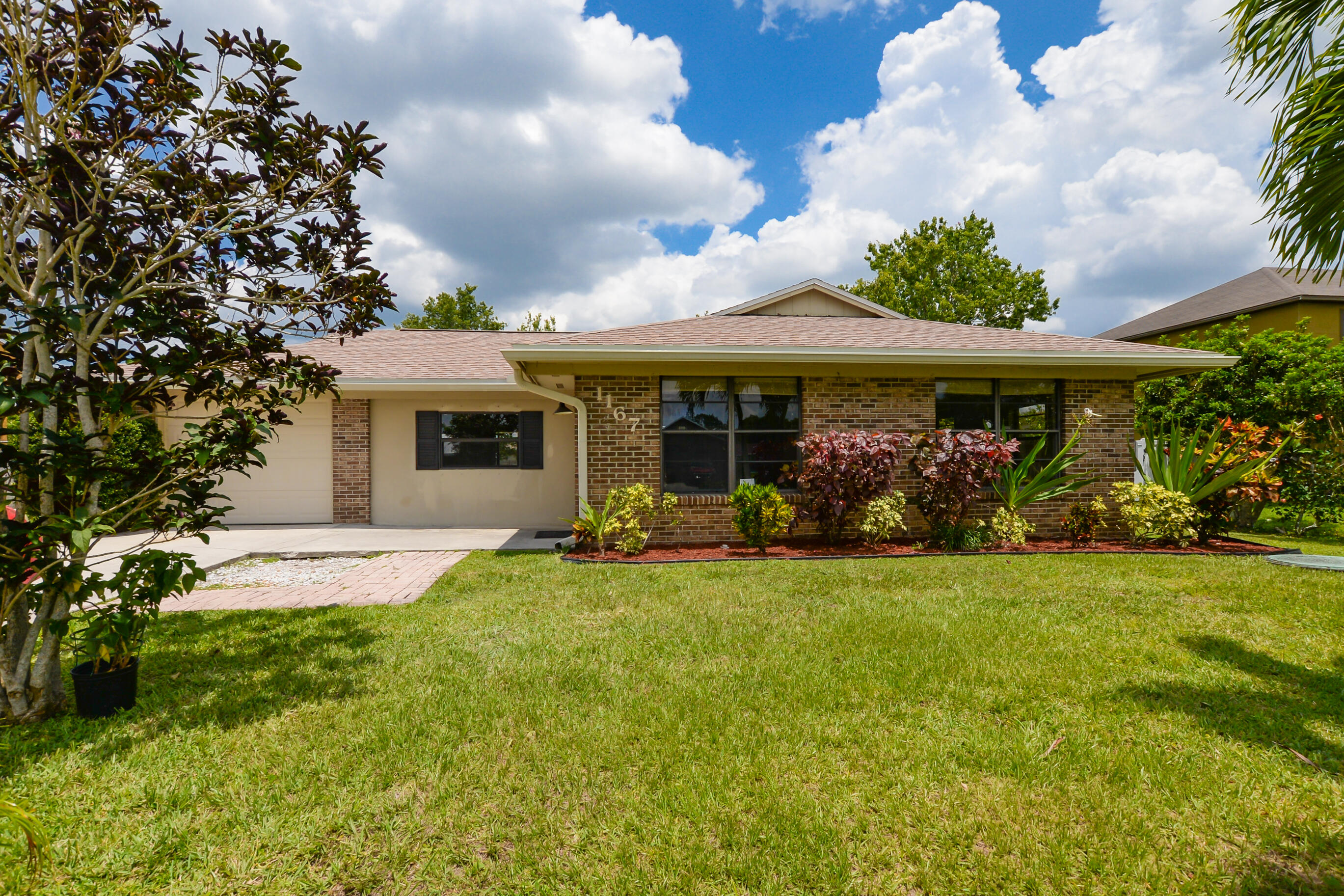This real estate photograph captures a charming single-story house, likely located in Florida or a similar climate, characterized by its brick and stucco construction. The front of the house features a brick façade, with brick trim extending to the rear wing, which includes a brick column flanked by stucco walls and a central window. The house also appears to have an attached garage with a concrete deck suitable for parking.

The well-maintained lawn is lush and green, bordered by a brick walkway leading from the driveway to the entrance. The front yard is landscaped with a planting bed filled with mulch, adorned with an array of shrubs—two of which are taller—and up to six smaller plantings, including palmettos or small palm trees. Among these are orange flowers and other tropical bushes, all surrounded by orange stones or bark chips.

A prominent tree stands at the front left corner of the property, accompanied by a potted plant. In the background, the bright blue sky is dotted with large cumulus clouds, underscoring the sunny day depicted. Additional details include the presence of a neighboring house, separated by a dense array of shrubs, and the presence of a palm tree frond visible in the upper right corner of the image. The architecture and landscaping suggest the house was likely built in the late 1970s or early 1980s.